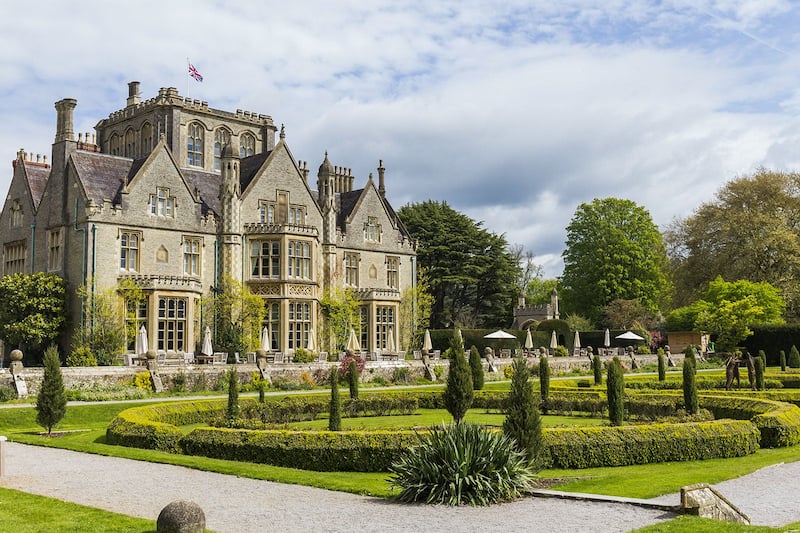This image features a large and stately country estate in England, characterized by its imposing stone architecture reminiscent of a small castle. The estate, with a resemblance to the Biltmore in North Carolina, boasts a rich architectural style with many tall chimneys and spires, numerous arched, peaked windows, and intricate roof lines. The front façade of the castle includes a grand entrance, possibly dating back to the Victorian era or earlier, showcasing extensive glasswork and stone masonry.

Surrounding the castle is a meticulously maintained classical English garden, adorned with boxwoods and cypress trees. The garden layout includes a distinctive circular driveway and garden area, where short, neatly trimmed bushes encircle taller trees, creating a protective yet picturesque scene. The front garden area is accentuated with tables and chairs, all shaded by numerous umbrellas, suggesting that the estate might now function as a hotel or a restaurant, providing ample seating for guests.

The backdrop features tall, mature trees, adding to the serene and majestic ambiance of the scene. The presence of a British flag flying atop the estate reiterates its location within the United Kingdom. The overall setting is serene and elegant, with the onset of spring bringing life and color to the garden and landscape, enhancing the visual grandeur of the estate.